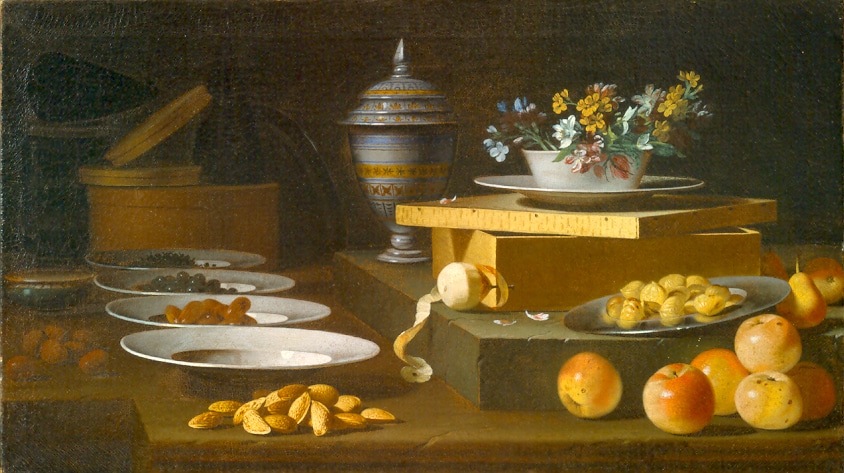This horizontal still life painting depicts an intricate tabletop scene, predominantly in various shades of brown, giving it a rich, earthy tone. The background is a dark brown wall, providing a stark contrast to the medium brown wooden table in the foreground. On the left side of the table, there is a row of white ceramic plates filled with assorted fruits and nuts, with one plate being empty. The items become increasingly complex towards the right side of the image.

On the right, the table has multiple elevated surfaces. A darker brown block serves as a base, holding a silver plate with pieces of yellow substance and various fruits, including apples and pears. A peeled apple sits on this block, with its peel cascading down to the main table surface. Above this block, a further wooden platform elevates a white plate containing a bowl filled with delicate flowers in shades of yellow, white, and blue.

A gray second-level structure supports this assembly, and behind it, a silver vase with colorful patterns and a pointy lid adds to the scene's vertical elements. Surrounding these central features, scattered elements include hat boxes and other obscure dark items subtly blending into the background. The careful arrangement of these objects, combined with the play of light and shadow, makes for a detailed and visually engaging composition.